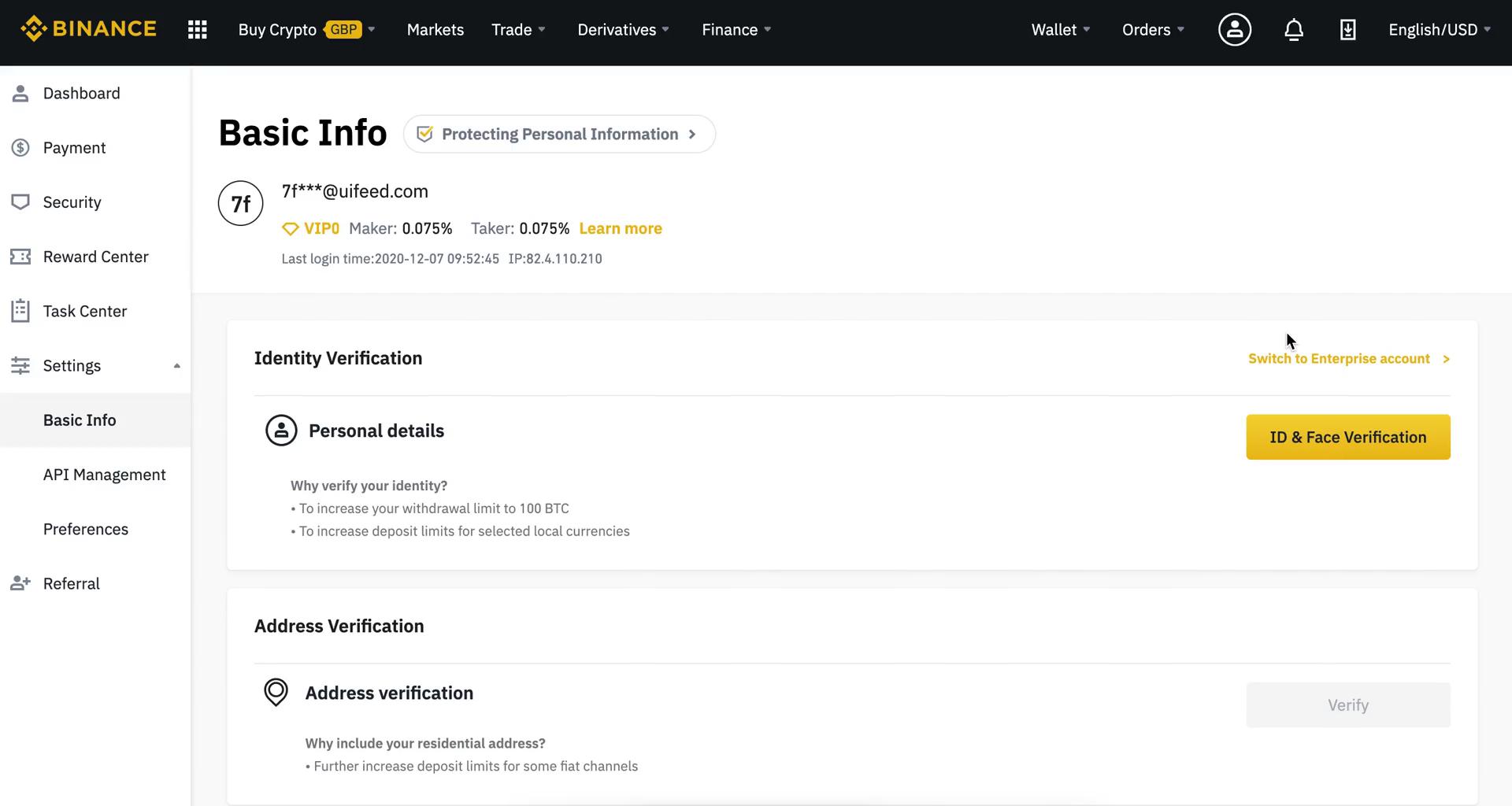The image appears to be a screenshot of a Binance user interface from a computer. The topmost section features a black header with "Binance" prominently displayed in yellow text on the upper left. Adjacent to this label, there's a 3x3 grid of small white dots. To the right of the grid, the text "Buy Crypto" is shown next to a yellow button labeled "GDP." Further right, additional menu options include "Markets," "Trade," "Derivatives," and "Finance." Continuing along the header, options for "Wallet" and "Orders" are also visible, alongside a bell icon and a language/currency selector displaying "English/USD."

On the left side of the interface, a vertical menu displays various folders: "Dashboard," "Payment," "Security," "Rewards Center," "Task Center," and "Settings." The "Settings" section is expanded to reveal subsections: "Basic Information," "API Management," "Preferences," and "Referral," with "Basic Information" currently selected.

Central to the screen is a panel titled "Basic Information," featuring a website URL, "7F at UIFeed.com." Below, there is a section labeled "Identity Verification" containing "Personal Details," with adjacent information on "ID and Face Verification." Above this section, a search icon is situated just above the "Switch to Enterprise Account" option.